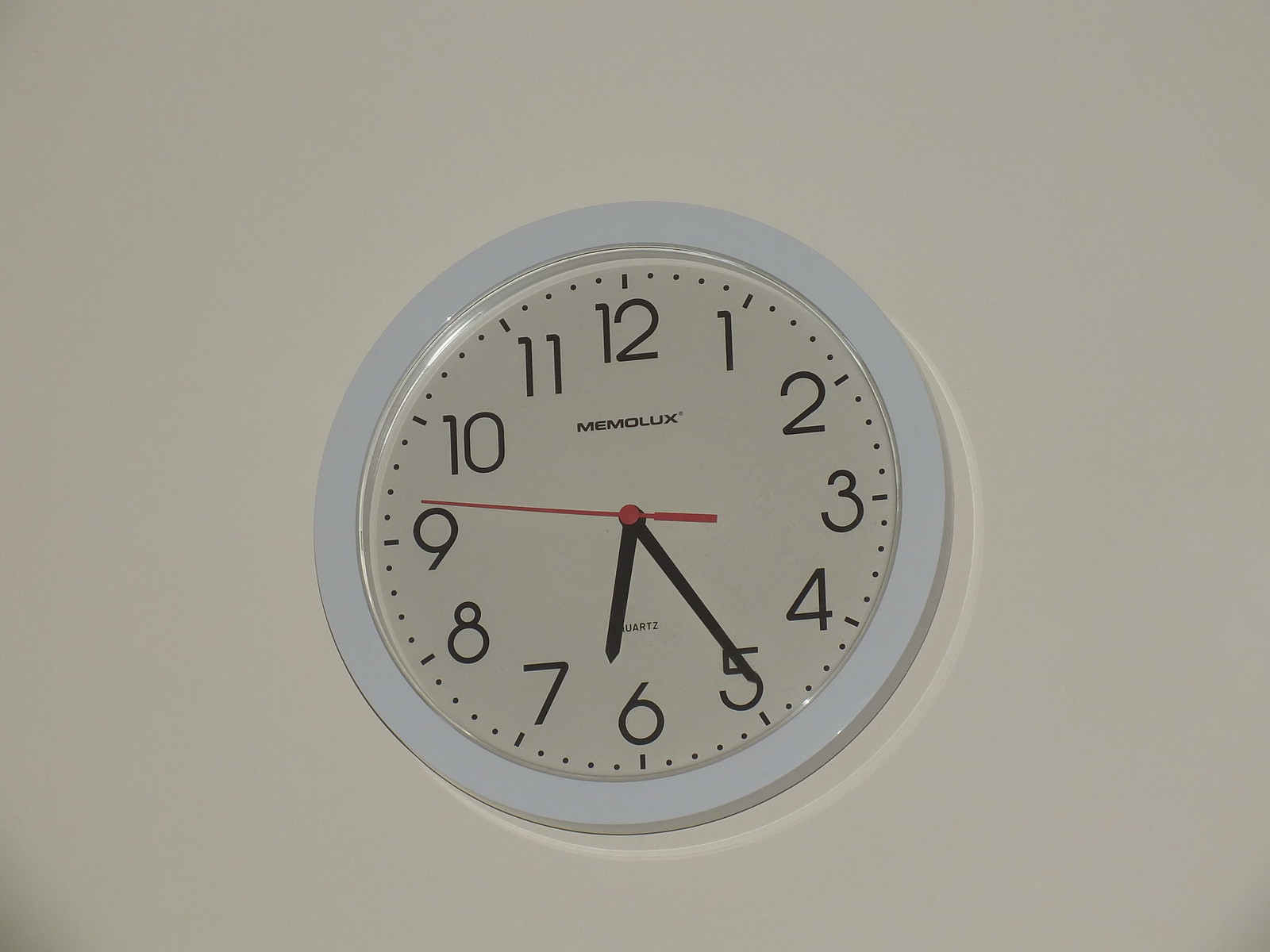A clean and detailed caption for the image:

"A minimalist clock is prominently mounted on a pristine white wall. The clock's circular face is also white, harmonizing with the wall behind it. There's a subtle reflection of light visible on the wall, forming a faint whitish ring around the clock. The brand name 'MEMOLUX' is printed in black font on the white clock face, just below the 12 o'clock mark. The word 'Quartz' is inscribed above the 6 o'clock position. The clock features two black hands and one red second hand, all set against black numerals that clearly denote the hours. Small black dots encircle the white clock face, marking the minutes. A light reflection can be seen on the protective covering of the clock face, emphasizing its clarity. The image is crisp and sharply focused, with no other objects present in the scene."